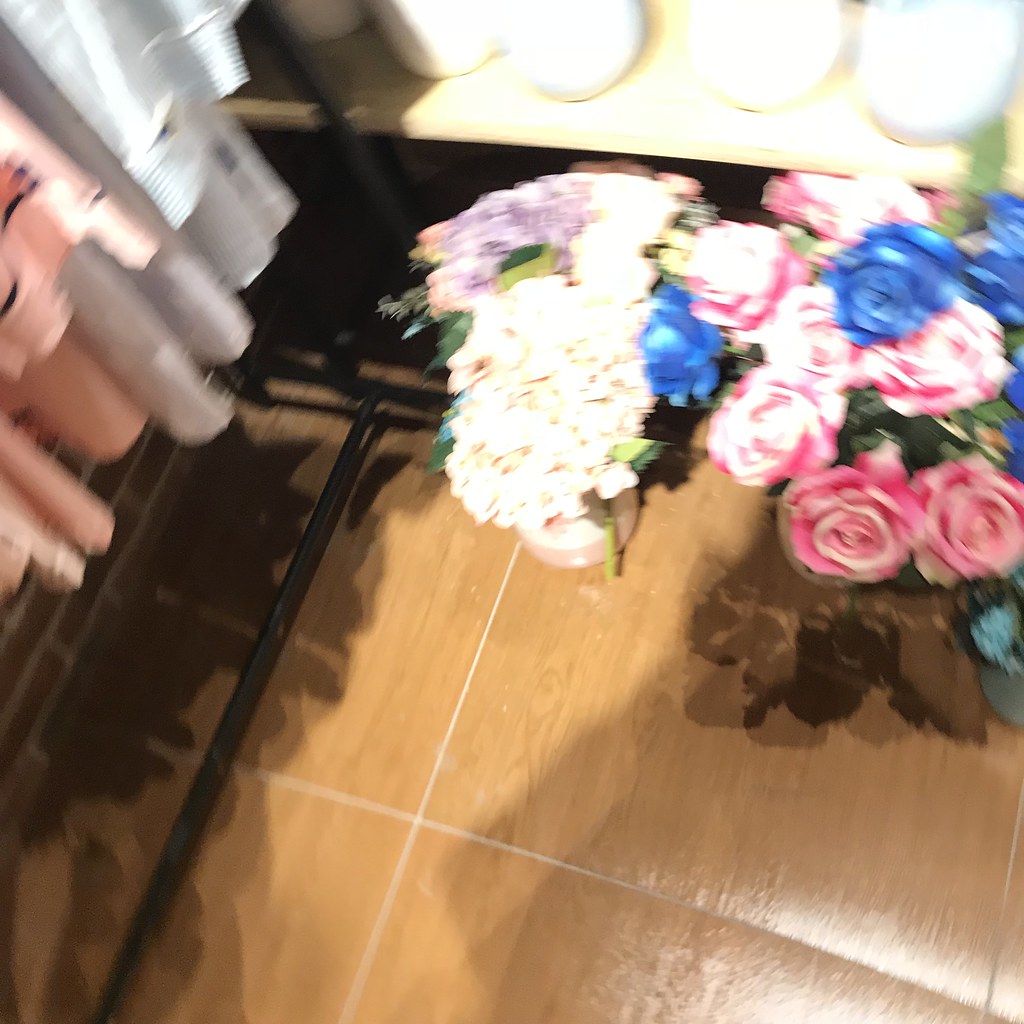In this slightly blurry image, we see what appears to be a flower shop with a detailed assortment of floral arrangements and various objects. The foreground features a wooden floor with distinct grains and lines, possibly accentuated by brown tiles with lighter grout. Multiple bouquets of flowers are arranged at the bottom, showcasing a colorful mix, including white flowers with purple accents, pink roses, blue flowers, and yellow flowers. 

To the left, there is a rack or possibly a rolling stand holding clothes, including silk or satin dresses in shades of pink and silver. Above, a pink vase with white flowers is visible, next to a bunch of violets, arranged on a tan wood shelf. This shelf also holds some brightly illuminated objects that look like candles, though their details are not entirely clear. 

On the right side of the image, there’s a visible mix of pink, blue, and purple flowers, complemented by green foliage. Furthermore, there is a black stand housing more pink and gray objects, adding to the room's diverse array of textures and colors. Despite the image’s lack of sharpness, the scene clearly depicts a vibrant, flower-filled space, likely a flower shop.